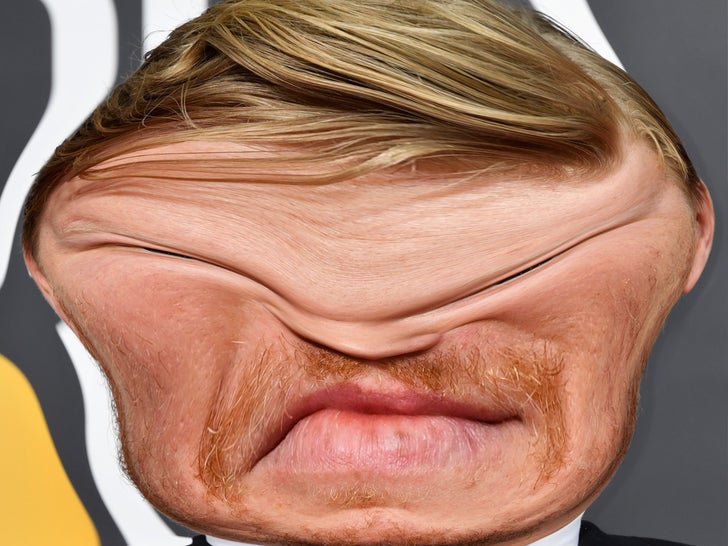The image depicts a close-up photograph of a white male with blonde hair styled longer on top and short on the sides. He has a reddish-orange mustache and stubble, with pink lips that appear slightly chapped. However, the man's face is heavily distorted, likely through digital manipulation or a filter, resulting in a smashed and deformed appearance. The forehead seems folded down, obscuring the eyes entirely and merging the nose with the eye area, giving his face an almost alien-like shape. The ears are exaggerated and visible only in parts. The man is dressed in a black suit with a white button-down collared shirt. The background is predominantly gray with scattered white and yellowish-orange lines, concentrated more toward the left corner.